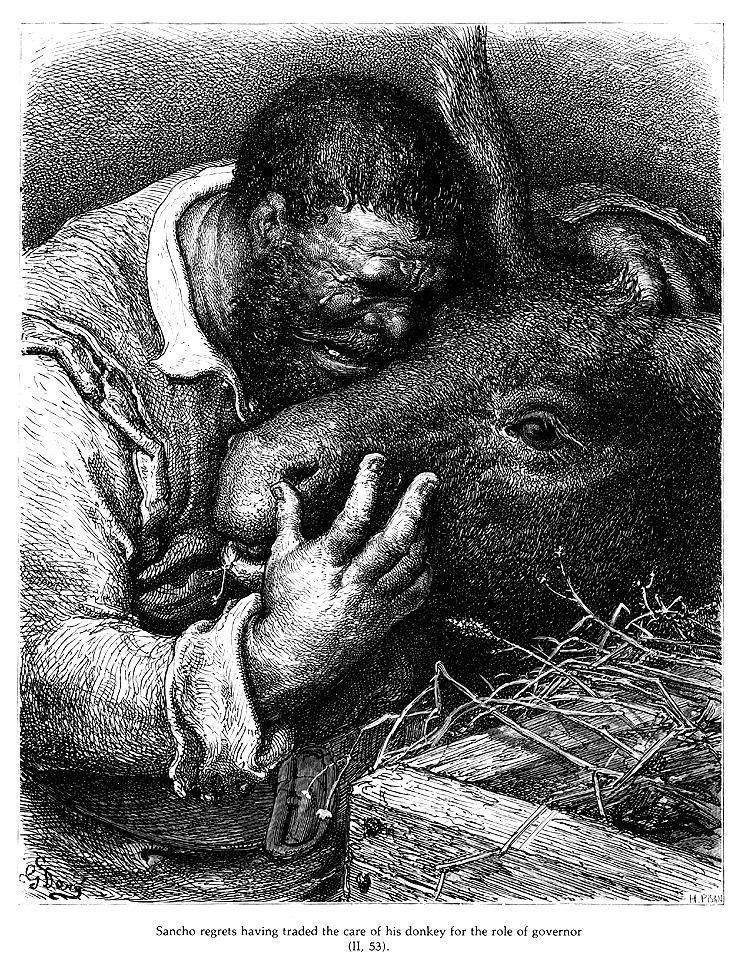The image appears to be an illustration, possibly from a book like Don Quixote, featuring a distressed man embracing the head of a donkey. The man has short black hair, a beard, and a mustache. He is dressed in a worn, long-sleeved shirt with a folded back sleeve and a white collar, along with a vest. His face is crumpled in sorrow, with a visible teardrop indicating he is crying. The man’s arm is wrapped around the donkey's face, and his head is buried against the donkey’s head. In the bottom right corner of the image, there is a box covered with straw. The artwork is rendered in grey and white tones and includes text at the bottom: "Sancho regrets having traded the care of his donkey for the role of governor (IL, 53)." The composition suggests a barn setting, emphasized by the presence of straw.